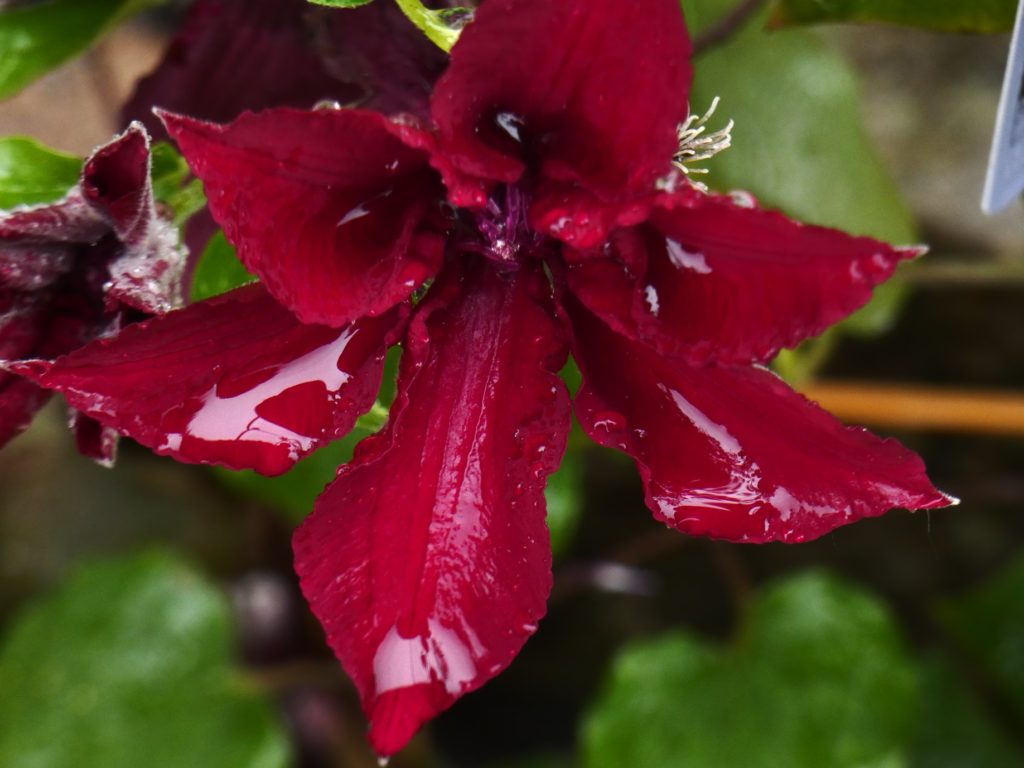This vibrant close-up color photograph captures a striking red flower as the central focus. The flower has six elongated red petals that are delicately tipped with light white, each glistening with water droplets, possibly from a recent rain. The petals, approximately three inches long, extend outward from a darker red-hued center adorned with a ring of central stems. Off to the left, there is an unopened bud, a darker red than the main flower, adorned with a subtle white fuzz at its base. In the upper right corner, a white tag hangs from a leaf, adding a unique element to the composition. The background features a mix of green leaves, some sharply in focus while others remain a pleasing blur, providing a lush, natural setting. This scene, bathed in hues of green, red, and hints of white and brown, suggests an outdoor garden environment, possibly during a rain shower.